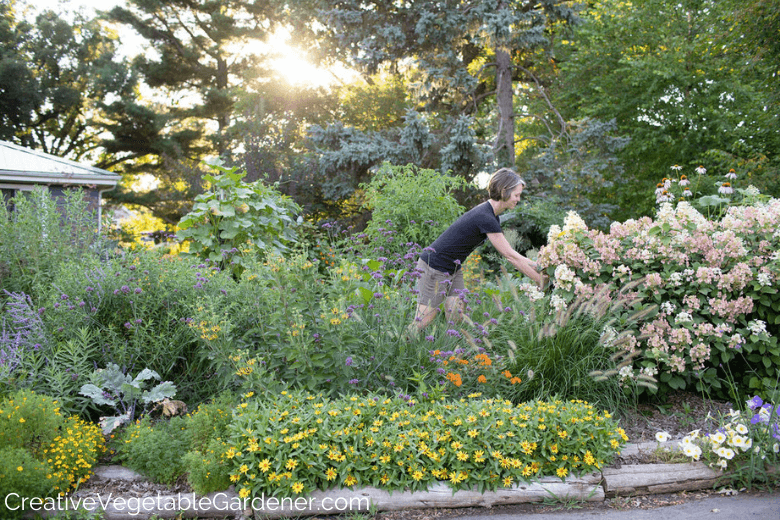The image, taken outdoors on a sunny day, captures a lush, verdant garden scene. In the square, full-color photo, a middle-aged Caucasian woman with short, graying brown hair is the central focus. She is engaged in gardening, tending to one of the flourishing flowering plants. Dressed in a blue t-shirt and khaki shorts, she appears to be picking blooms. Surrounding her is a plethora of plants, some flowering in vibrant hues of yellow, white, and purple, with others showcasing rich green foliage.

The garden, thriving with both deciduous and evergreen trees, gives a strong sense of summertime. Log barriers delineate the garden space, adding a rustic charm. Although the garden seems to be part of a larger residential area, possibly along a road or driveway, it lacks any distinct background. A hint of a building, which might be her house, is visible. The top-left section of the image captures the sun peeking through the dense canopy of trees, providing a softly illuminated ambiance.

At the bottom-left corner of the image, there is a watermark: "CreativeVegetableGarden.com," although vegetables are scarce, with possibly only a hint of kale among the predominantly floral and green landscape.